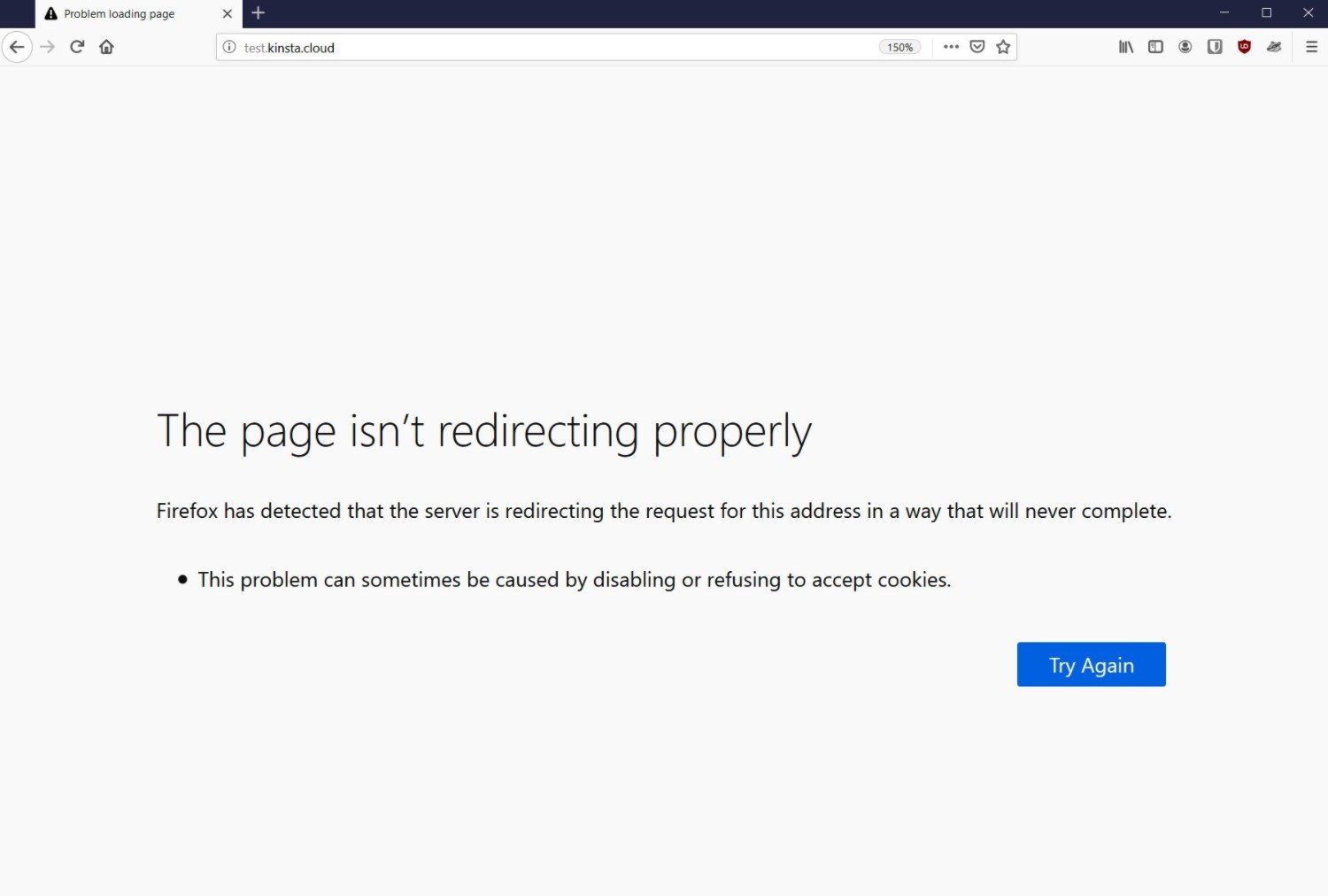Screenshot of a webpage attempting to run a test on **test.kinsta.cloud**:

- **Background**: Gray.
  
- **Top section**:
  - **Black bar** at the top.
  - **Pop-up warning** on the left with a black triangle and an exclamation point, reading: "Problem loading the page".

- **Toolbar** (beneath the black bar):
  - Left arrow, right arrow, refresh button (circular arrow), and home button.
  - **Search bar** with the text "test.kinsta.cloud".
  - At the end of the search bar: 
    - Zoom level of "150%",
    - Three dots (menu),
    - Check mark,
    - Star.
  - On the far right: Six icons including books and profile.

- **Main content**:
  - **Error message**: 
    - Text: "The page isn't redirecting properly".
    - Additional information: "Firefox has detected that the server is redirecting the request for this address in a way that will never complete. This problem can sometimes be caused by disabling or refusing to accept cookies".

- **Right-hand side**: 
  - Blue pill button with white font saying "Try Again".

The detailed visual elements and error messages provide a comprehensive insight into the issue encountered while attempting to access the test webpage on **test.kinsta.cloud**.